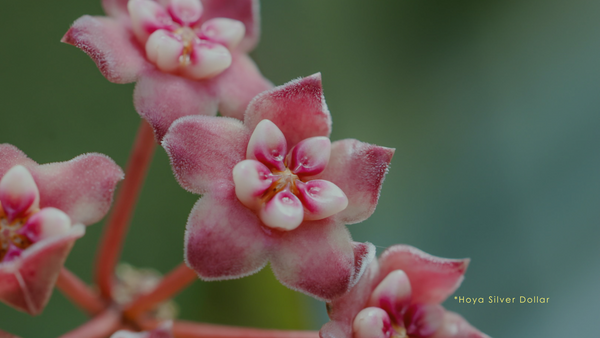This close-up image features a cluster of delicate flowers identified as Hoya Silver Dollar, denoted in small yellow text with an asterisk or dot to its left, located in the lower right corner. The background is an out-of-focus green, perhaps indicating trees or leaves, giving prominence to the foreground. The flowers exhibit a unique structure with five interconnected petals that create a seamless appearance. These petals transition in color from a softer pink near the center to a richer purple towards the tips, with fuzzy, soft edges. Central to each flower is an intricate arrangement of shiny, round, tooth-like white projections, adorned with magenta, converging to a yellow core. The stems showcase a reddish hue, adding contrast to the pink and white of the petals. The detailed close-up reveals four flowers connected to a single base, with an additional stem extending beyond the image frame. The overall composition of the flowers, with their fuzzy petals and tooth-like centers, creates a surreal and oddly enchanting visual.